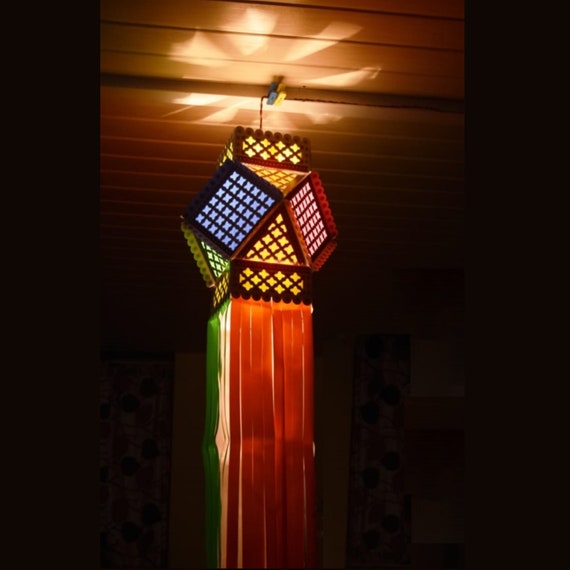The photograph captures an intricately designed, multicolored Asian-style lantern hanging from a ceiling made of tongue-and-groove wood panels. The image is in full color and vertically oriented, with the lantern suspended by a small chain. The lantern features an octagonal shape with panels of blue, red, yellow, green, and gold, each adorned with small square holes that allow light to filter through. The top sections of the lantern are triangular, while the middle sections are square, forming a complex 3D design that resembles an eight-sided dice. The lantern emits a soft, warm glow that illuminates the immediate area, accentuating the various colors and intricate detailing of the panels. Hanging from the bottom of the lantern are long, flowing streamers in red, green, and white, which extend to the lower edge of the photograph. The overall surroundings are pitch black, emphasizing the lantern as the focal point of the image.